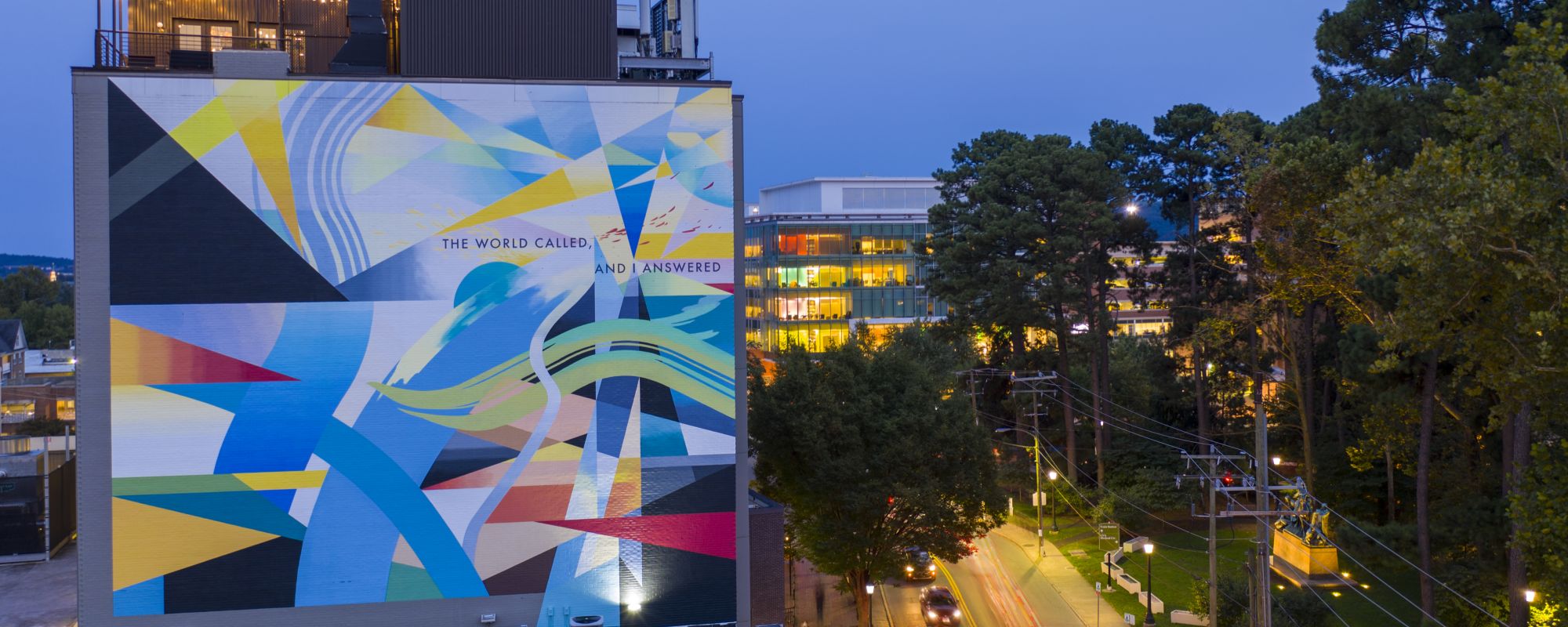The image captures an urban landscape at dusk or dawn, featuring a prominent tall building on the left-hand side adorned with an abstract mural in shades of blue, yellow, red, and black. The mural includes geometric patterns of triangles and swooshes and features the text, "The World Called and I Answered." This artistic piece spans the side of the building with a small patio visible above it. In front of this building, we see a scene with power lines, telephone poles, and men working on the wires, alongside a yellow cable car. Below, cars with headlights on travel along a lit street. In the background, another tall building stands with its windows all illuminated, indicating an active evening. To the right of the scene, there are trees and a park area, adding a touch of nature to this cityscape. The overall lighting suggests it is either early morning or late evening, as the sky is light yet the streetlights and building lights are glowing brightly.